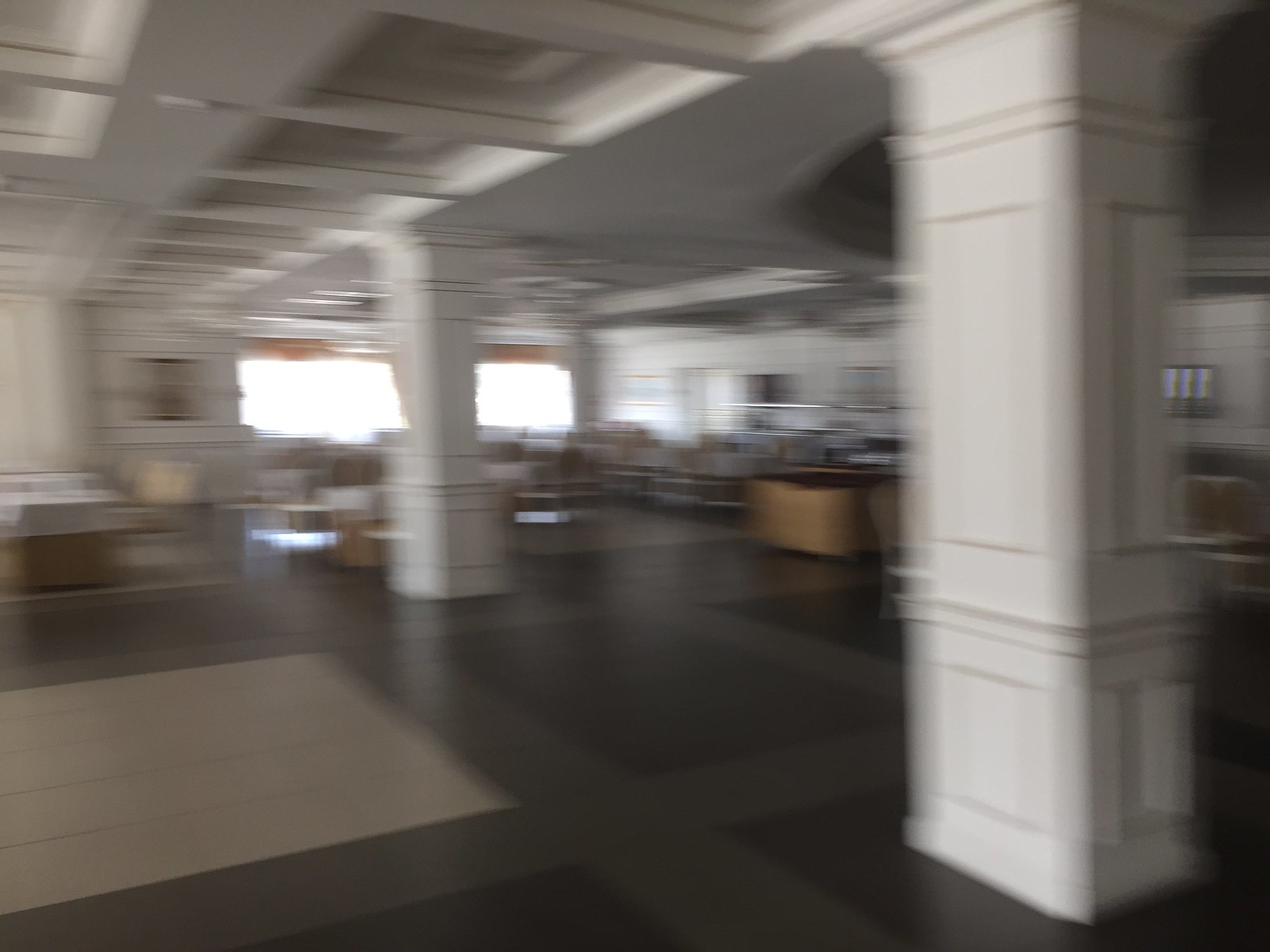This photograph, though very blurry as if taken mid-motion or by mistake, captures the interior of an elegantly designed room. The flooring is a detailed pattern of black or dark brown squares, intersected by dark gray striped walkways and a patch of light gray tile on the left side. In the center stand two white rectangular pillars adorned with intricate carvings, contributing both to the room's stability and aesthetic appeal. The room contains brown tables and chairs, mostly visible in the background, where a large, bright, white-lit window with brown curtains enhances the light. The ceiling, painted gray, completes the sophisticated ambiance of the space.